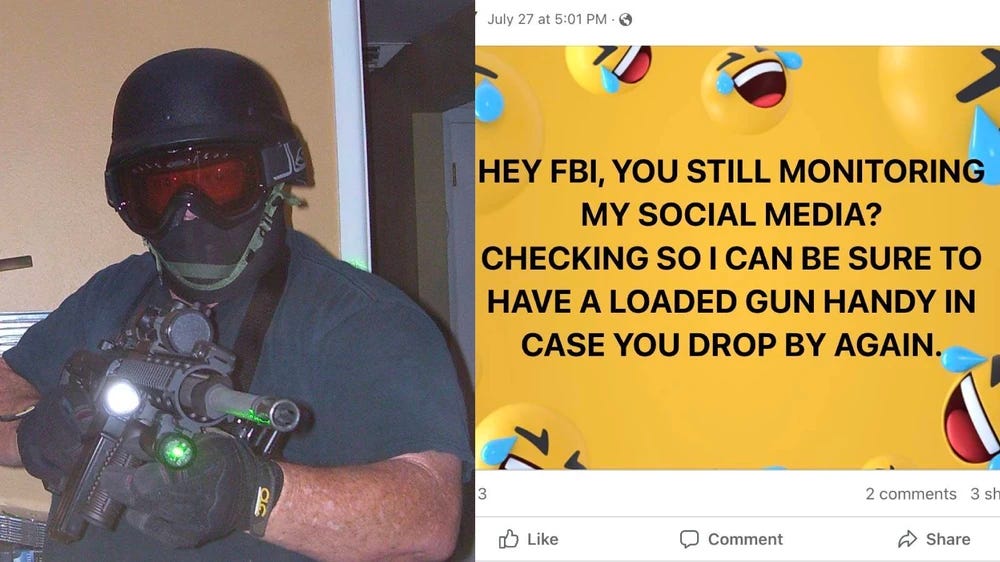The left side of the image features a man dressed in riot gear. He wears a short-sleeved blue t-shirt that exposes his arms, paired with a metal helmet that covers his forehead and extends down the back of his neck. He also sports red goggles and what appears to be a mask covering the lower part of his face, possibly part of the helmet. A green strap band is visible, and he is holding what looks like a machine gun emitting white and green lights. His hands are encased in black gloves. The background suggests he is inside a house.

On the right side of the image, there's a yellow rectangle with black fonts that reads: "Hey FBI, you still monitoring my social media? Checking so I can be sure to have a loaded gun handy in case you drop by again." Surrounding this text are various laughing emojis, crying with laughter. Below this message, it indicates "two comments, three SH," and includes options for like, comment, and share, timestamped July 27th at 5:01 pm. The predominant color of this section is a school-bus yellow. Despite his gear, the man's lack of body armor makes him appear less intimidating, somewhat resembling an accountant due to his outfit.